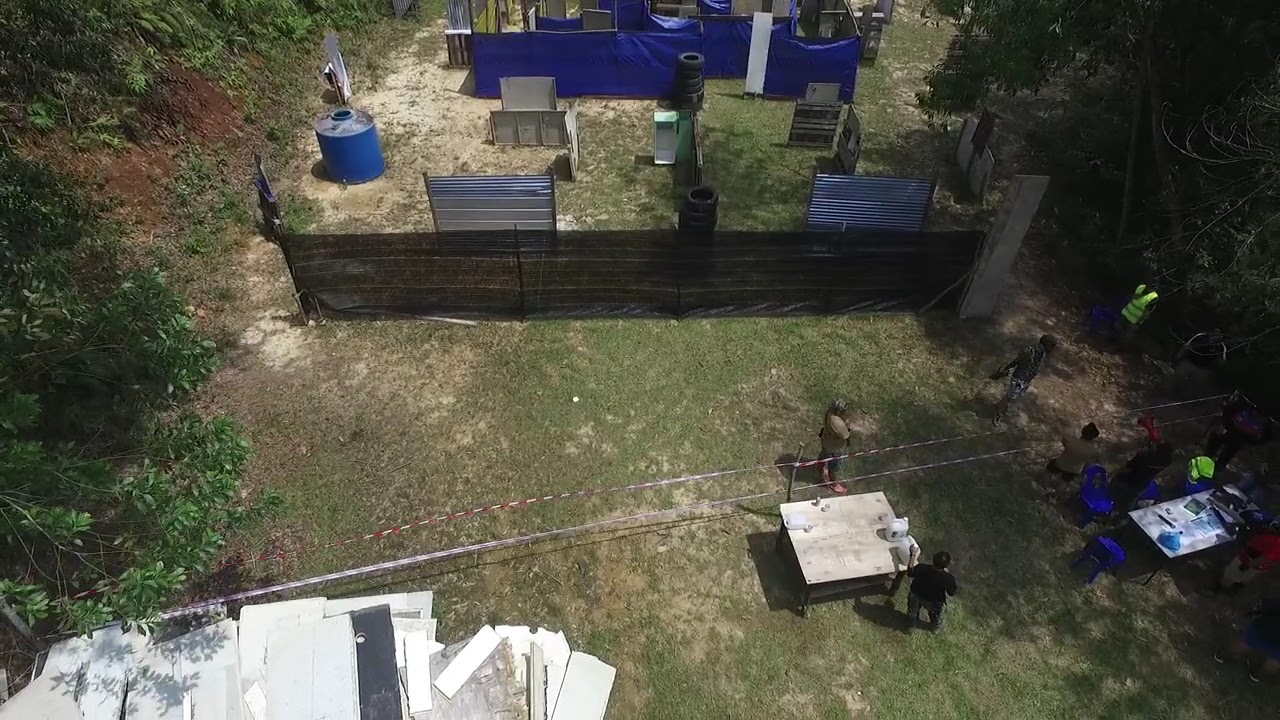The image, taken from a high vantage point, shows a grassy yard interspersed with patches of dirt, segmented by various colored tarps. A prominent black tarp, supported by posts, stretches across the center. Beneath this tarp, people are gathered around a gray-colored table. To the right, strong shadows partially conceal two individuals in bright neon green vests. 

Further in the background, two sets of silver steel barriers stand, with additional blue tarps stretched across them, contributing to what resembles an obstacle course. In the upper left of the image, a dirty blue barrel with a narrow opening can be seen. At the bottom left corner, a pile of what appears to be roofing slabs is scattered. The presence of plans laid out on the tables and pieces of wood to the side suggests an ongoing work activity, possibly constructing or setting up a structure. Trees frame the scene on both the left and right sides of the image.